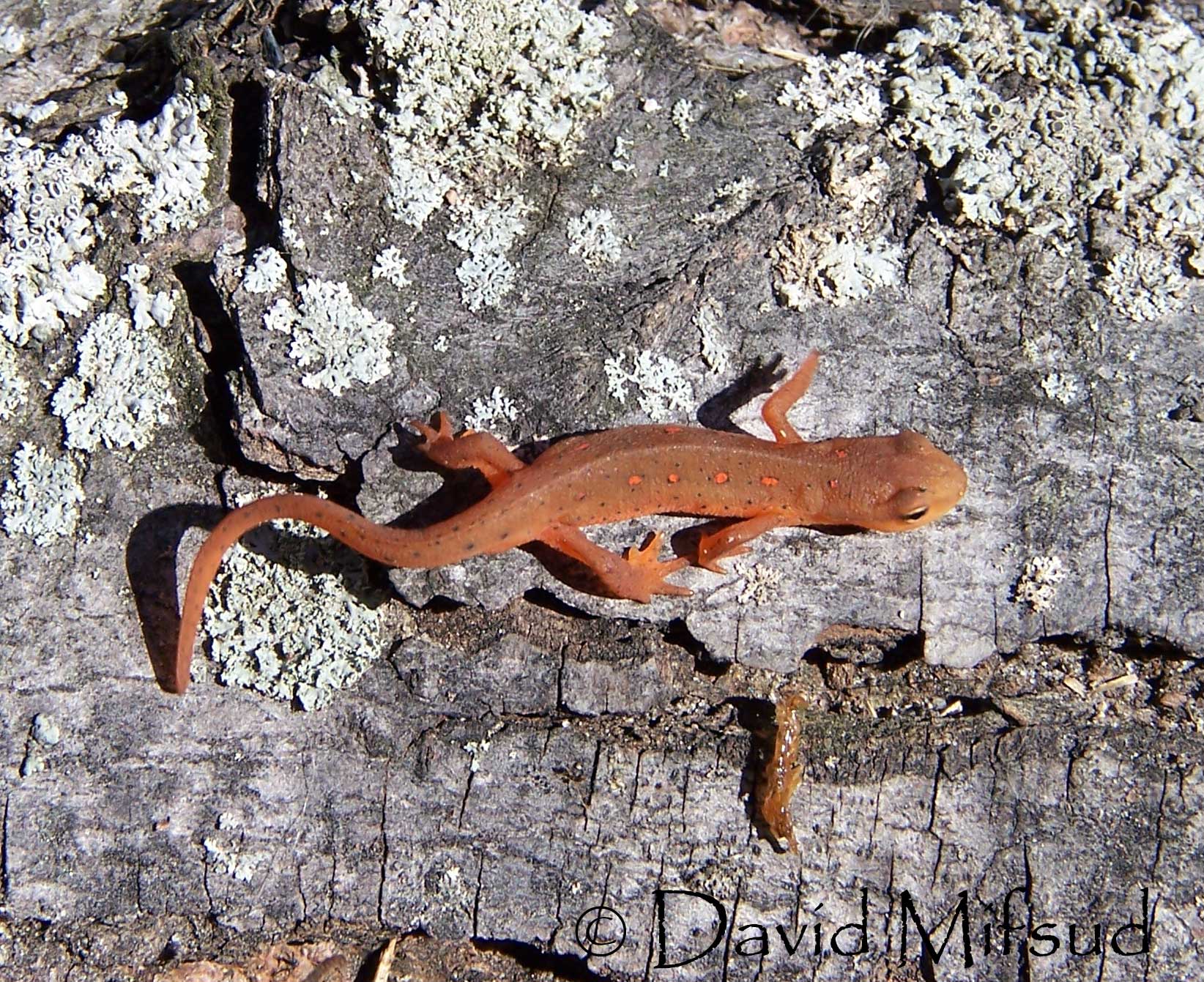This photograph, taken outdoors from a top-down perspective, features an orangish-red lizard with distinct coloration and patterns. The lizard's body is adorned with dark spots, with larger dark spots particularly noticeable on its tail. Along its back, near the spine, are brighter orange spots that create a striking contrast. The lizard’s eyes are dark, and its nose is a lighter shade than the rest of its body. Positioned on a primarily gray, slightly brownish piece of tree bark that has patches of light green, almost white, moss, the lizard is in the center of the frame, crawling towards the right. The bark has a textured surface with flowering speckles, enhancing the natural setting. Below the lizard, there is a smaller creature, resembling a snail. In the bottom right corner of the image, the text "David Misfood ©" is visible, indicating the photographer.